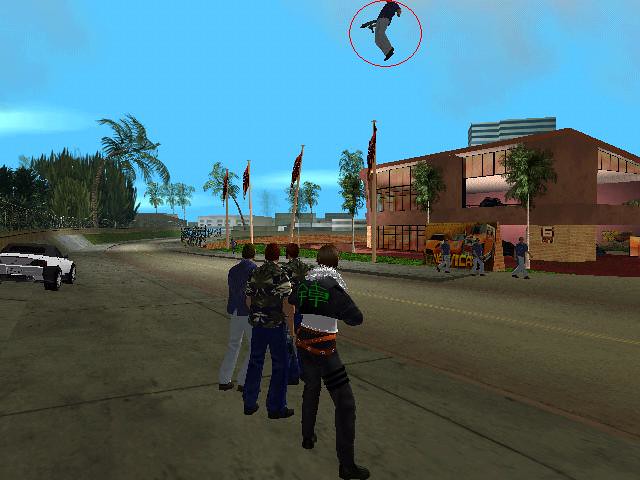This image is a highly pixelated, likely modded in-game screenshot reminiscent of older video games. The scene features a gray concrete sidewalk flanked by a grayish asphalt road with a yellow line in the center, creating an urban setting. On the left side, there's a white sports car with a black roof and black wheels parked near a building that resembles a white sports bar. Across the road on the right side, there's a light tan and reddish brick building marked with a number '6', and further back, several white buildings can be seen. Palm trees and various flags line the street, adding to the vibrant atmosphere. 

In the foreground, there are four male characters, some possibly modded, with one bearing a striking resemblance to Squall from Final Fantasy 8. They are dressed in diverse outfits, including blue jeans, an orange belt, a camouflage shirt, and khaki pants. 

Dominating the upper part of the image, a man floats in mid-air, encircled by a red marker to draw attention. He is clad in khaki pants and a dark shirt and wields what looks like an Uzi machine gun. The sky is a baby blue with scattered white clouds, completing this bustling and chaotic in-game street scene.